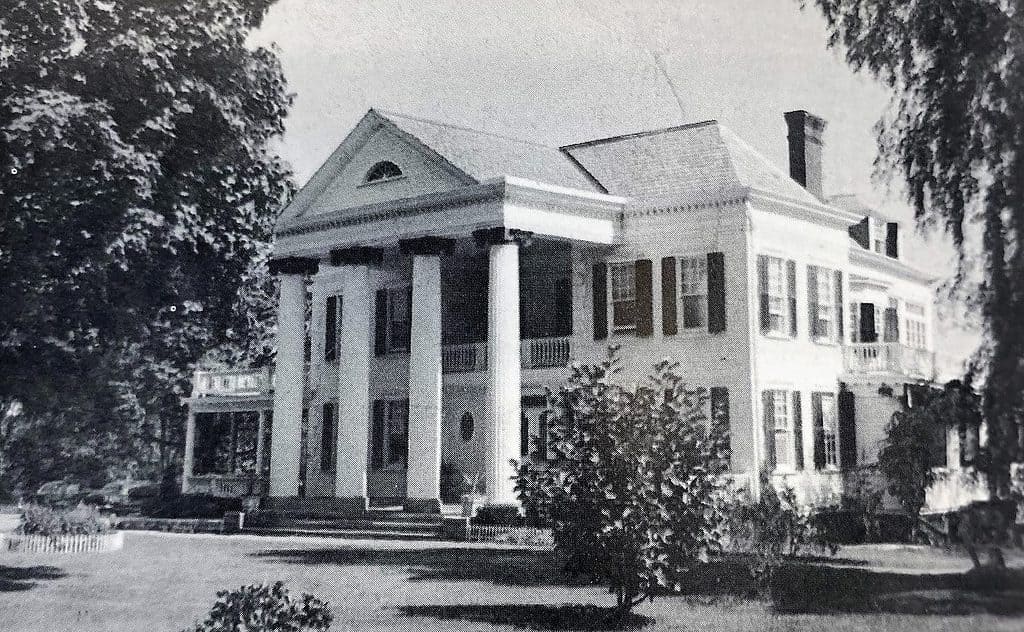This black-and-white photograph captures a large, colonial-style mansion that exudes an air of historical grandeur. The two-story structure features four prominent, white stone columns at its entrance, reminiscent of classical architecture, perhaps similar to the entrance of the White House. The columns, with their striped design and pedestal tops and bottoms, support a slanted roof that houses a semicircular attic window. Below, the well-manicured lawn showcases a small tree to the front, framed by larger trees on both the far left and right sides.

The mansion includes multiple windows spread across its facade, with some featuring shutters. A balcony and an upper-level deck add to the house's intricate design, along with a stone or brick chimney located towards the back. The front yard features a roundabout driveway, enhancing the suburban feel that is evocative of neighborhoods like those depicted in "Leave it to Beaver" or "Mayberry." The grainy quality of the photograph, likely due to its age, introduces a nostalgic charm, while the sky remains indiscernible due to the image's monochromatic nature.